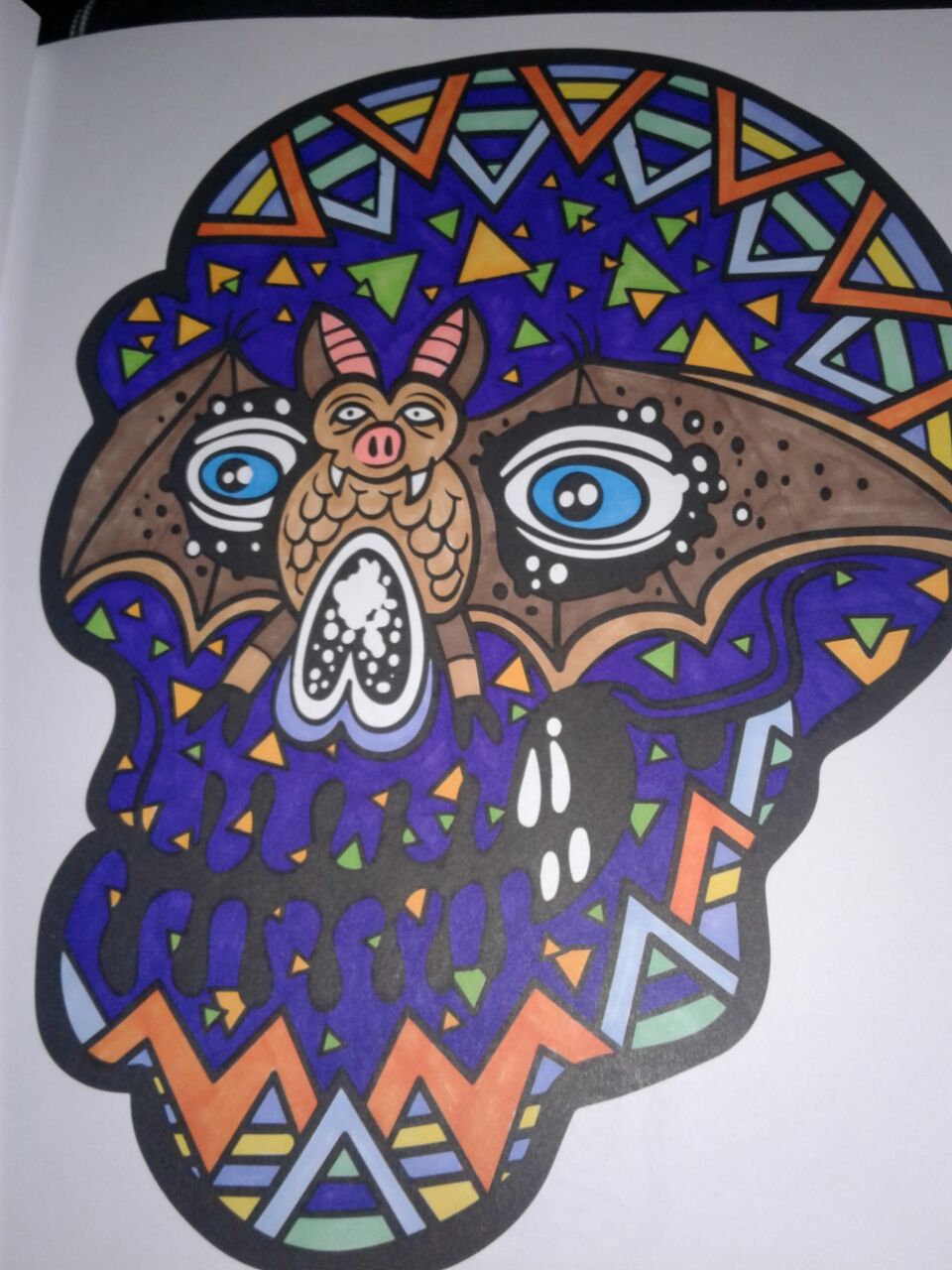The image is a detailed, vivid drawing of a multicolored skull filled with various geometric shapes and designs. The skull features small spaced teeth and a prominent bat positioned just above its nose cavity. This bat, which is brown with white accents, has its wings extended around the eyes of the skull, creating the illusion that the eyes are within the bat's wings. The background of the skull is primarily dark blue and black, adorned with an assortment of green, yellow, and orange triangles. These triangles are scattered across the forehead, mouth area, and chin, creating a zigzag pattern that extends from the chin to the top of the skull. Additionally, a light blue triangle with green, blue, yellow, and light blue stripes is visible at the bottom of the design. The entire image is set against a light gray background, making the vibrant colors and intricate details of the skull's design stand out even more.